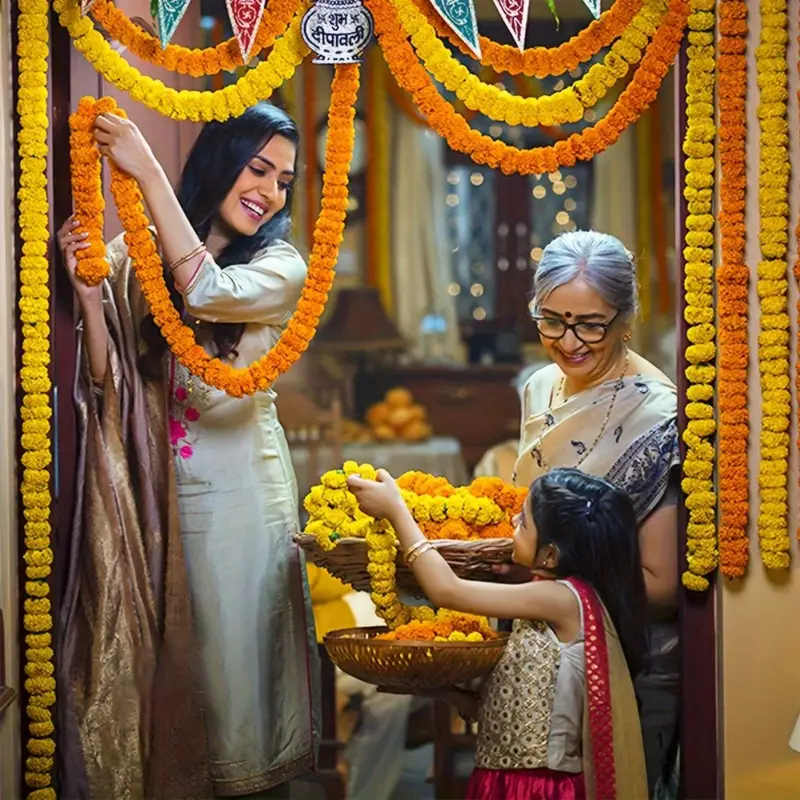The photograph captures a vibrant moment of three generations of Indian women decorating the doorway of their home with colorful ornamentations. The scene is set in what appears to be the kitchen, at the doorway, where two women and a young girl are engaged in festive preparations. 

The eldest woman, possibly in her 60s or 70s, with gray hair pulled back in a bun, wears glasses and a purple and white sari adorned with intricate ornamental designs. She has a traditional dot on her forehead and a warm smile as she looks down at her granddaughter. She holds a basket filled with decorative items.

The younger woman, seemingly in her 20s or 30s, has long black hair and is dressed in a white, richly embroidered Indian dress. She is smiling down at the young girl, holding an orange, puffy lei-like decoration, about to hang it over the doorframe. 

The young girl, with long dark hair pulled back from her face, is dressed in a gold-embroidered vest and a pink skirt. She holds another basket filled with similar decorations and offers one to her mother. The decorations, which resemble bright yellow and orange plastic leis, hang from the doorframe in alternating colors, creating a lively, celebratory atmosphere. The shared task and mutual smiles suggest a joyful family moment, rich with tradition and intergenerational bonding.